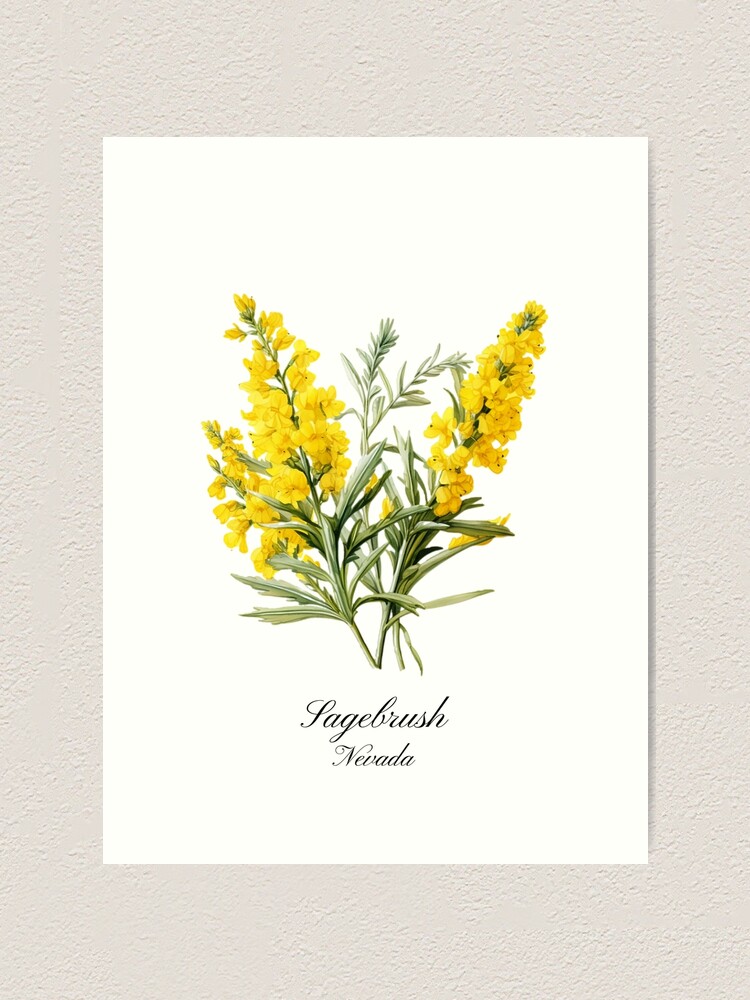The image depicts a framed card featuring an illustration of Nevada sagebrush. The card, made from a high-quality white cardstock paper, showcases three vibrant yellow flowers with small clustered petals that contrast beautifully with their long green stems and leaves. The yellow blooms, distinctly emerging from slender green stalks, somewhat resemble tiny yellow ducks with small black specks that look like eyes. Below the floral illustration, elegant black cursive text labels the plant as "sagebrush," followed by "Nevada" underneath. The framed card is displayed against a white stucco-finished wall.